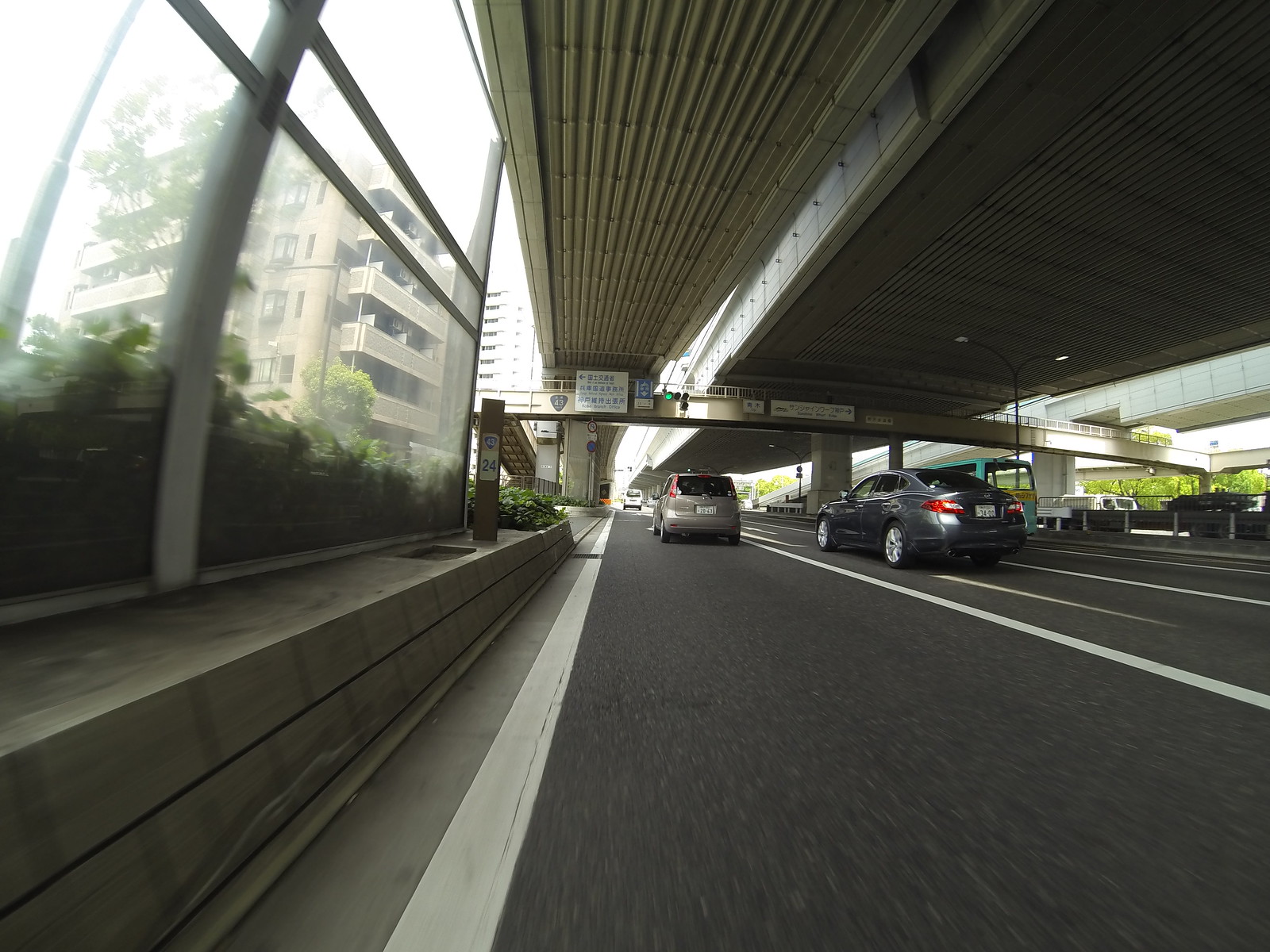This photograph captures a bustling urban scene where vehicles navigate a road beneath intersecting bridges. In the upper left-hand corner, a white building with balconies stands against a backdrop of a gray, overcast sky. To the left of the image, a concrete Jersey barrier-like island separates the road from a section with lush plants visible through a plexiglass barrier.

On the roadway, clear solid white lines demarcate the lanes. In the left lane, a tan minivan progresses, while a gray sedan drives in the right lane. Overhead, the underside of two bridges is visible, characterized by white concrete strips running along their lengths. Additionally, a footbridge spans horizontally across the center of the photo, adding to the complex layers of infrastructure in this urban environment.